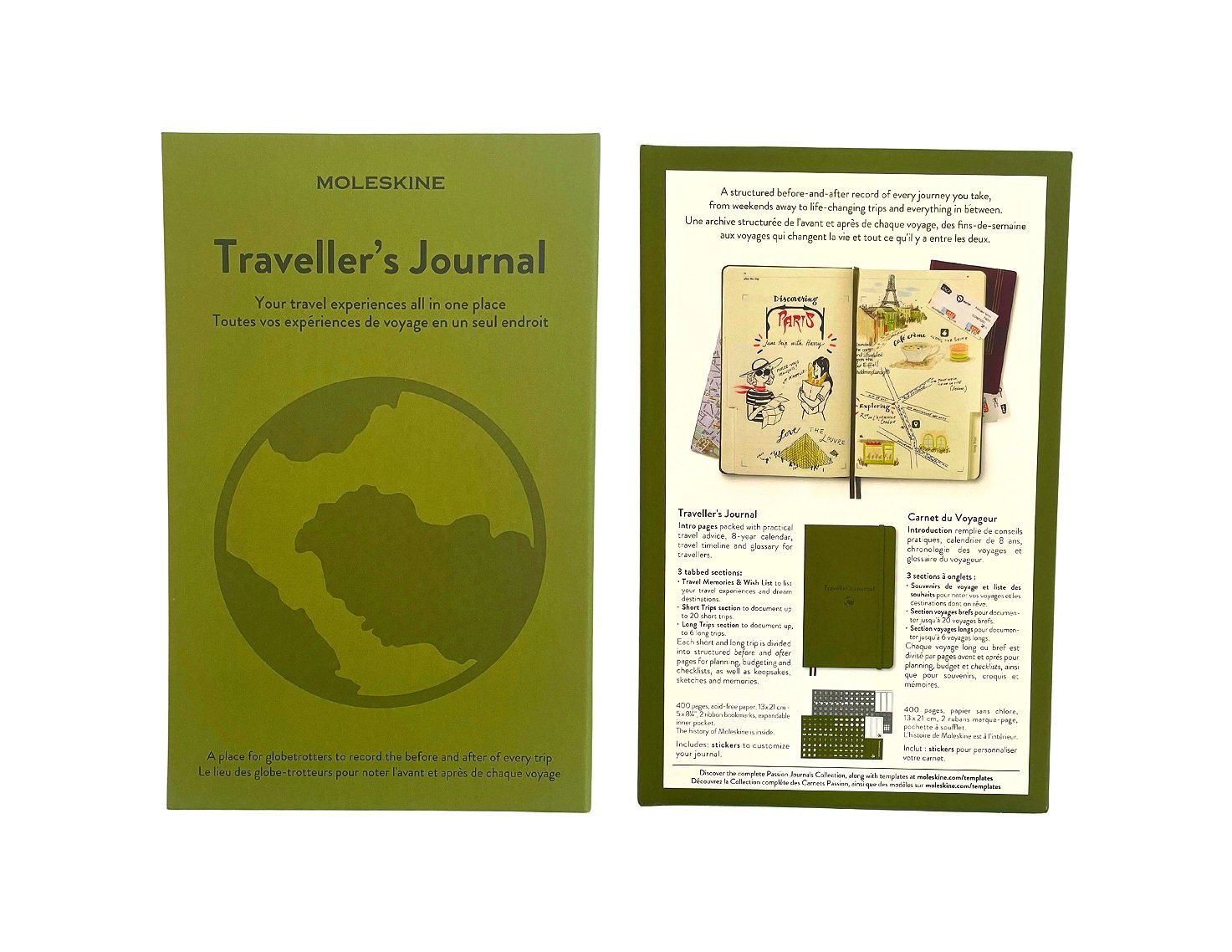The image depicts two views of a Moleskine Traveler's Journal. The first view showcases the journal’s cover, which is made of green leather or moleskin, featuring the title "Traveler's Journal" and the phrase "your travel experiences all in one place" printed in dark green lettering. Beneath this, the same phrase appears in another language, possibly French. At the center of the cover, there's a rough illustration of a globe highlighting several continents. The second view presents the journal when opened. It contains various texts and illustrations, including travel maps and drawings of people, on a white background framed in deep olive green. The detailed layout suggests it may have areas dedicated to documenting travel experiences, although it is unclear if it includes pockets for items like a passport.